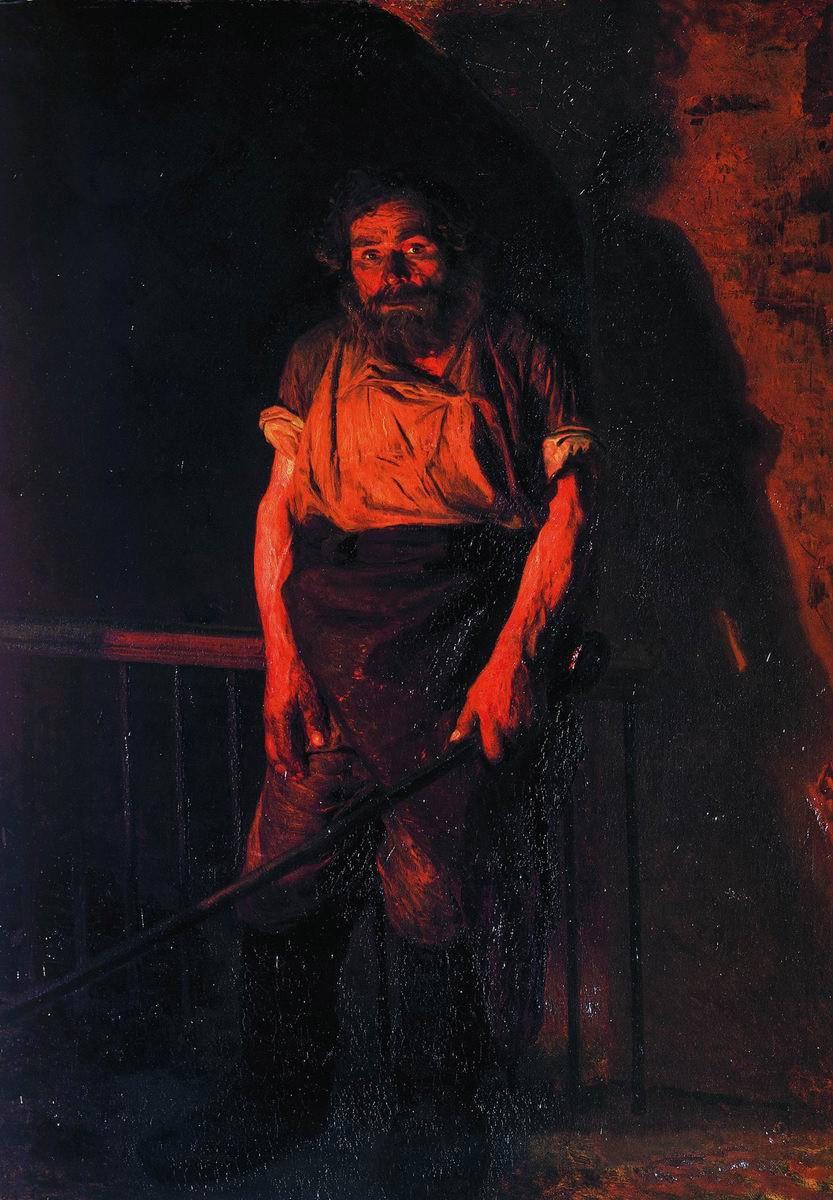This evocative painting depicts an older man, possibly a blacksmith or tradesman from the 19th century, standing in a dim, almost night-like scene. The overall atmosphere is dark, with his figure dramatically illuminated by the reddish glow of what appears to be a nearby fire, casting a stark shadow behind him. The man has very dark hair, a full beard, bushy eyebrows, and a mustache, all distinctly highlighted by the light's glow. He is dressed in old clothes, including an apron-like garment over his pants and a shirt with the sleeves rolled up, revealing veined and muscular arms that suggest a life of labor. His hands and face have traces of what appears to be soil, adding to his rugged appearance. In his left hand, he holds a long, black pole, which could be a tool or even a fishing pole. Behind him is a railing with steel supports, and possibly a tree over his shoulder. The scene is bathed in an ominous red light reflecting off a smooth wall behind him, enhancing the sense of him being at work, potentially in a forge. The man gazes directly at the viewer, creating a powerful connection within the dark, moody setting.